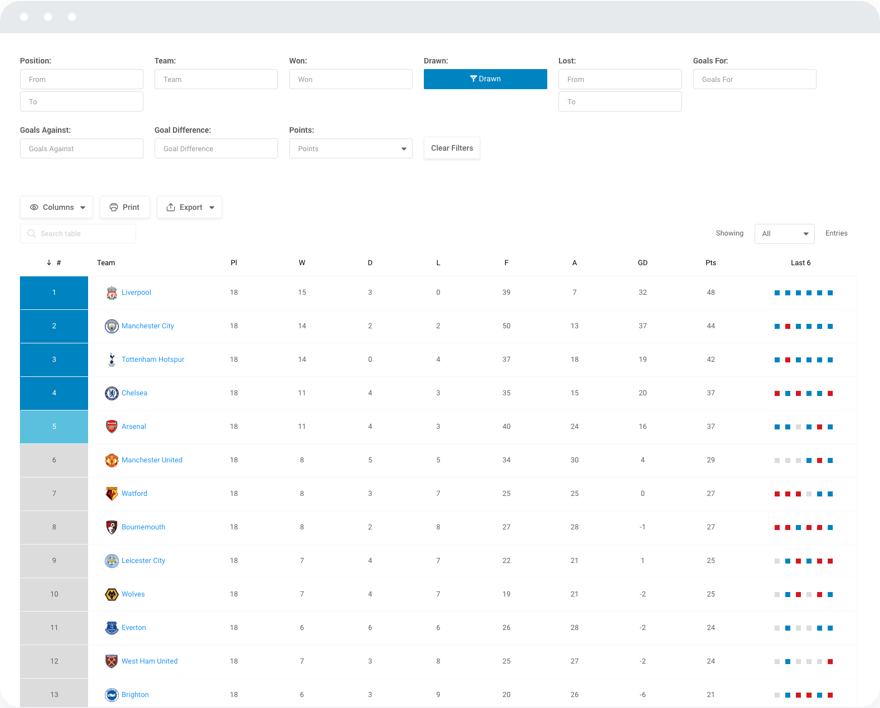The image features a structured table/chart often used for data sorting and filtering within a software application. The top portion of the image has a light gray background with three white circles located in the upper left-hand corner. Below this, the background transitions to white.

At the top, the word "Position:" is written in black with a colon followed by two outlined gray boxes labeled "from" and "to". Adjacent to this is another gray outline box marked "Team:", with the corresponding label "Team 1." Below this, a row contains an outlined gray box stating "Draw:", followed by a teal-colored rectangular button featuring a white funnel icon and the word "Draw" in white. The next row includes a similar area labeled "Lost:" outlined in gray, along with several white rectangles of gray borders labeled "from" and "to".

Underneath these filters, the table header lists various categories: "Goals For:", "Goals Against:", "Goal Difference:", and "Points:". Each category has matching rectangular fields with gray borders containing the respective category titles in gray font. 

At the bottom of the table headers, there's a white rectangle with a gray border, containing the text "Clear Filters" in black. Just below this, there is a row of action buttons labeled "Columns," "Print," and "Export."

Additionally, the table appears to list team statistics, evidenced by the labels "P", "W", "D", "L", "F", "A", "GD", "Pts", and "Last 6". Below these headers, the table displays the message "showing all entries".

On the left side of the image, a vertical row of colored boxes is visible; the first four are blue, while the fifth is light blue.